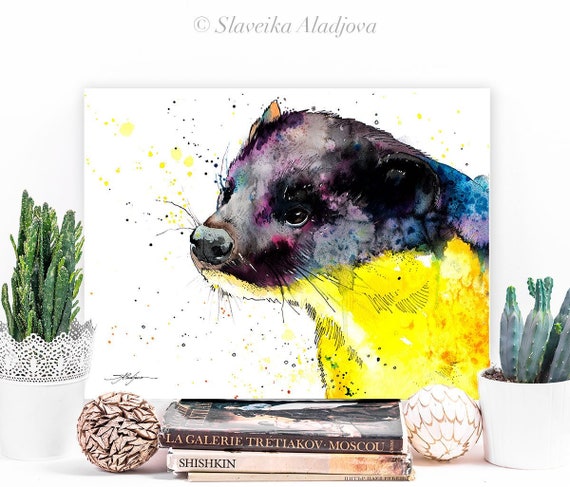The image depicts a vibrant watercolor painting of what appears to be a sea otter or ferret, prominently featuring lifelike proportions and intricate details. The animal, with its curious expression, is portrayed in a close-up, emphasizing its nose, eyes, whiskers, and ears. The painting combines realistic outlines with splashes of color; purples and blues blend with dark blacks and grays, while neon yellow and orange highlight its chin and underbelly. Surrounding the painting are paint splatters on a white background, adding an artistic flair. The scene includes two small cacti flanking the painting, which rests on a stack of art books with titles including “La Galerie Tretyakov, Moscow” and “Shishkin.” In front of the books are two paper balls, and the entire setup suggests a potential product photo from the Slovakian artist Ladová, whose name along with "copyright Slovakia" is visible on the artwork. The composition, rich in colors like yellow, purple, blue, and green, is likely set in a home, capturing a cozy and artistic atmosphere.